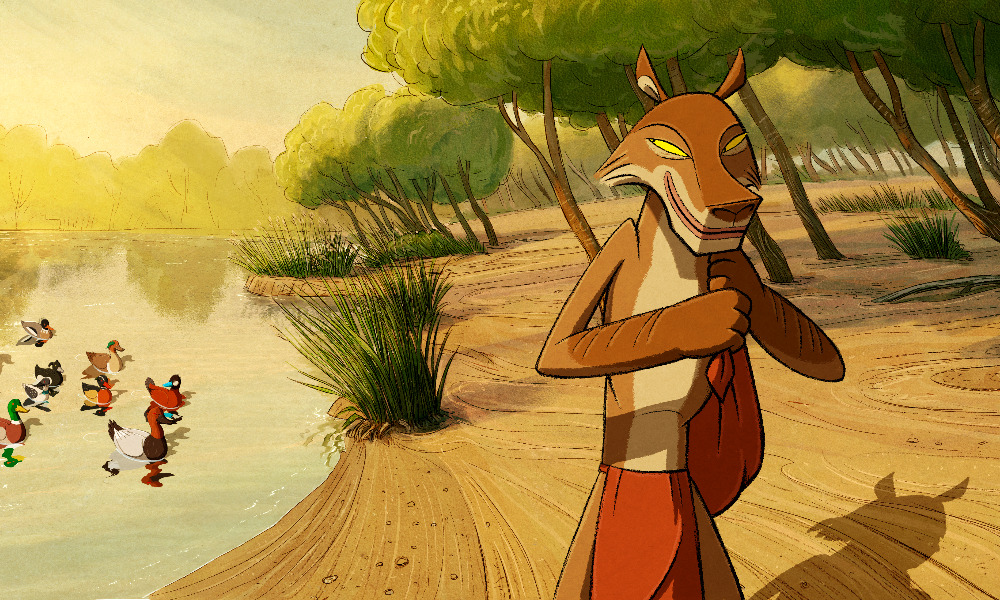The painting is a vibrant and detailed illustration, rectangular in shape, measuring about five inches wide and three inches high. It depicts a sunny day by a tranquil lake, with numerous colorful ducks floating on the still, cream-colored water. The ducks are a mix of green and brown mallards, red-necked, white-backed ducks, blue-billed ducks with red backs and brown heads, and other varieties, adding up to about eight in total.

On the right side of the painting, a cleverly anthropomorphized fox stands on its hind legs, casting a shadow to the right. The fox, brown in color, is adorned in red clothing and clutches a red bag, looking over its shoulder with a sly smile and yellow eyes, seemingly contemplating the ducks and possibly a nefarious plan. The fox's body language, along with its cunning expression, suggests a mischievous intent.

Surrounding the fox, tufts of tall green grass sprout from the brown sandy lakeshore. The landscape is dotted with green trees with brown trunks, encapsulating the serene lake scene under a clear blue sky. The overall style of the painting gives it an animated and whimsical quality, evocative of a scene from a children's cartoon or movie.